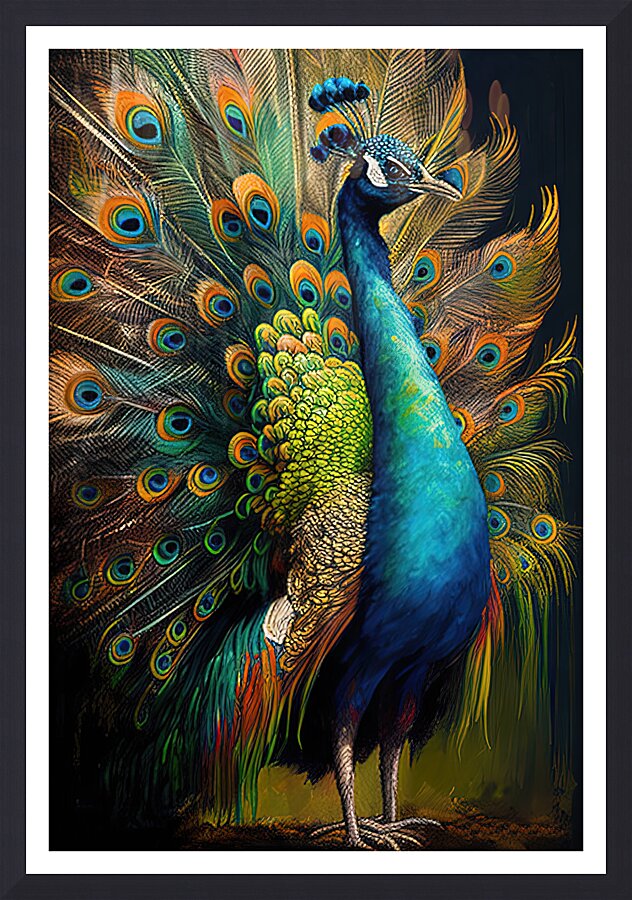This is a vertically oriented, rectangular image bordered by a thick black outline with a subsequent white inner outline. Within these borders lies a stunning and detailed depiction of a peacock, which appears to be a hand-painted or possibly computer-generated artwork. The male peacock is standing upright, facing right, showcasing its vibrant and elaborate plumage. The bird's body is predominantly blue, featuring gradations from dark blue on the head down to a brighter blue on the chest and belly. The peacock's head is adorned with deep blue feathers, complemented by blue plumes extending upwards, and a distinctive white patch immediately behind its eye. 

The peacock's beak is a tan color, and the bird stands on pale, almost cream-colored legs, which appear to be set on a dirt-like surface. Behind the bird's neck is a mix of green and tan feathers leading into the lush, fanned tail feathers. The expansive tail displays an array of vivid colors, including red, orange, yellow, blue, and green, each feather featuring 'eye' spots with a vibrant palette: orange on the outer rims with black and blue in the centers. The magnificent plumage stretches across the entire height and width of the image, although the very top of the tail is slightly cut off.

The overall impression is one of a colorful, almost neon brilliance, with the peacock's feathers creating an intricate pattern that captures the eye with its swirling layers and multi-colored spots. The artistic nuances in the depiction, such as the nearly lifelike texture of the feathers and the vibrant gradations of color, make this portrayal of a peacock both captivating and visually striking.